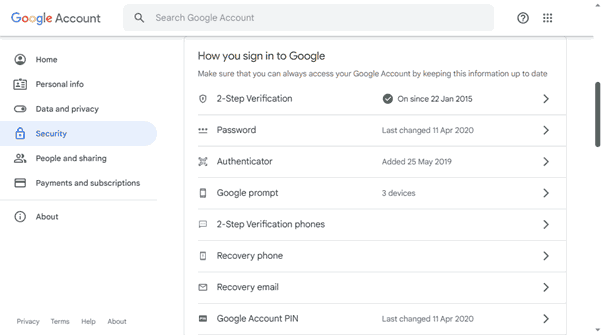Here is a cleaned-up and detailed caption for the image:

---

The screenshot depicts an email settings page from a Google account interface, set against a white background. At the top left, the Google logo is displayed with the capital "G" in blue, the first "O" in red, the second "O" in gold, the lowercase "g" in blue, the lowercase "l" in green, and the lowercase "e" in red. To the immediate right of the logo is a bold black text that reads "Account," encased in a rectangular box with a thin grey border and a mid-grey background. Within this box, there is a dark black magnifying glass icon and the text "Search Google account" in dark grey.

On the left-hand side, there is a vertical navigation bar with several tabs, each accompanied by an icon and bold black text:

1. A silhouette icon of a person in black with a semi-circle body, labeled "Home."
2. An icon resembling a newspaper with a person’s silhouette on the left, labeled "Personal info."
3. A slider icon with an oval shape and a black circle, labeled "Data and privacy."
4. A blue-bordered, rounded square icon with a lock, labeled "Security."

On the right-hand section, bold black text reads "How you sign in to Google," followed by regular black text: "Make sure that you can always access your Google account. Keep this information up to date."

Below this is a shield icon next to bold black text: "2-Step Verification." Adjacent to this, a black circle with a white check mark and the text "On since 22 Jan 2015." Each section listed below has a black arrow pointing to the right:

- "Password" (bold black) with details in regular black text: "Last changed 11th of Apr 2020."
- "Authenticator" with an X-like symbol: "Added 25 May 2019."
- "Google Prompt" with an icon of a cellphone and dark black text: "Used on 3 devices."
- "2-Step Verification Phones" with a chat bubble icon.
- "Recovery Phone" with a square icon featuring a black bezel.
- "Recovery Email" with a white envelope outlined in black.
- "Google Account PIN" with a dark black square background and white text, stating "PIN" in all caps. "Last changed 11 Apr 2020" in grey next to it.

Returning to the left-hand side navigation, more tabs are visible:

- An icon of two silhouetted people; the front silhouette is white, and the back is black, labeled "People & sharing."
- An icon resembling a credit card with a black magnetic strip, labeled "Payments & subscriptions."
- A dark black circle with a black eye in the center, labeled "About."
- At the very bottom in regular black text are the links "Privacy," "Terms," "Help," and "About."

---

This comprehensive description covers the layout and details of the email settings page from a Google account.